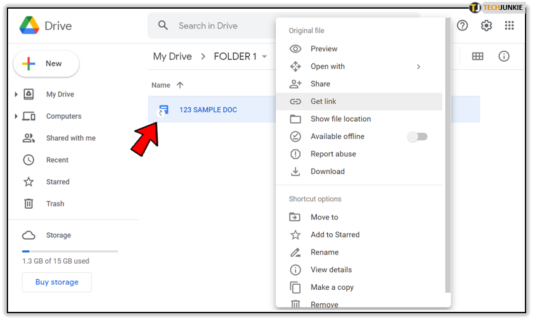The image displays a Google Drive interface brimming with features and options. At the top, a search bar allows seamless searching within the drive. Users can also pose questions or tweak settings. Adjacent to this are links to other Google services, notably Google Docs. 

The left sidebar is populated with several options: the ability to create new documents, access 'My Drive', sync with computers, view shared items, and check recent, starred, or storage status. Notably, the user has utilized only 1.3 GB out of the 15 GB available storage, with an option to purchase additional space. 

The main section is currently open to a folder named 'Folder 1', highlighting a document titled '123 Sample Doc'. Various actions can be performed on this document, such as previewing, opening with specific apps, sharing, generating a link, showing the file location, making it available offline, reporting abuse, downloading, moving, starring, renaming, viewing details, making copies, or deleting it. The user mentions familiarity with this setup due to its use at their workplace.